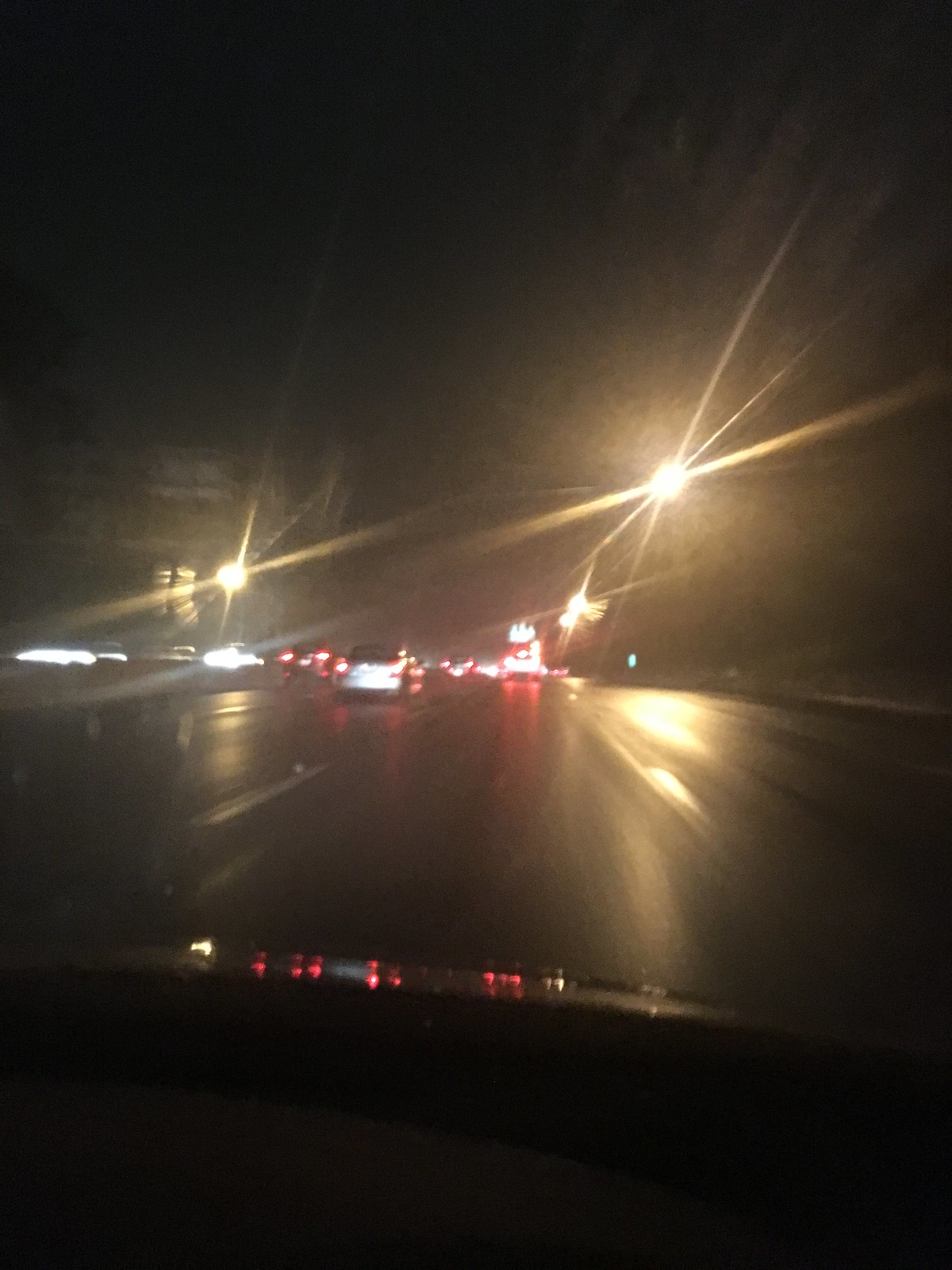This nighttime dash cam image captures a highway scene from the passenger side perspective of a moving car. The image is somewhat blurry, with a noticeable windshield glare adding to the effect. Ahead, several lanes span in both directions, separated by a small steel barrier. The highway is bustling with traffic; at least seven cars are visible in front, primarily four-door vehicles, identifiable by their red brake lights. The car in the foreground, likely a silvery metallic hue, has its hood partially visible. Streetlights on either side of the road cast a strong yellowish-orange glow, their light streaming outward and reflecting off the wet pavement, which imbues the road with an orange hue. Additionally, the brake lights of the cars create a streaming effect on the wet surface. Street signs are present on the right, and tall buildings with illuminated interiors can be glimpsed on the left, enriching the urban nighttime atmosphere.